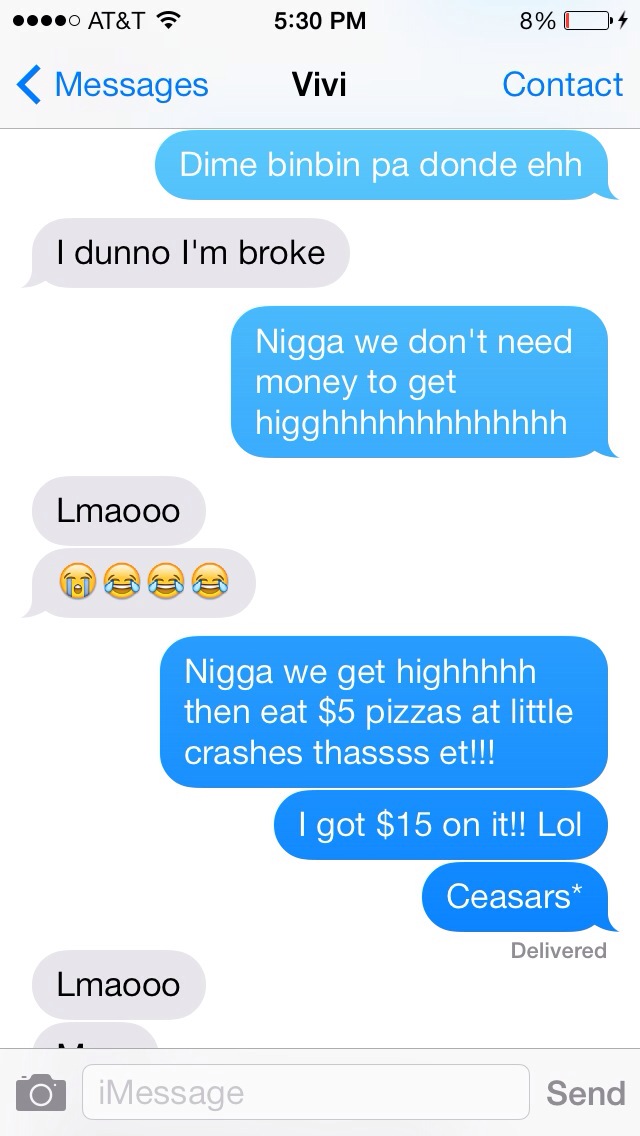This screenshot from an iPhone, displaying AT&T service at 5:30 p.m. with the battery charging at only 8%, captures a text message exchange between two individuals. The conversation, highlighted by alternating blue and grey message bubbles, begins with the sender texting, "Dime been been pa donde eh." The receiver replies, "I don't know, I'm broke," to which the sender responds, "Nigga, we don’t need money to get high." The receiver finds this amusing, replying with "LMAO" followed by several cry-laughing emojis. Continuing the discussion, the sender says, "Then we get high, then eat $5 pizzas at Little Caesars. That's it. I got $15 on it, LOL," correcting a typo from "Crashes" to "Caesars." The receiver once again responds with "LMAO." The screenshot ends with the text input box visible at the bottom.